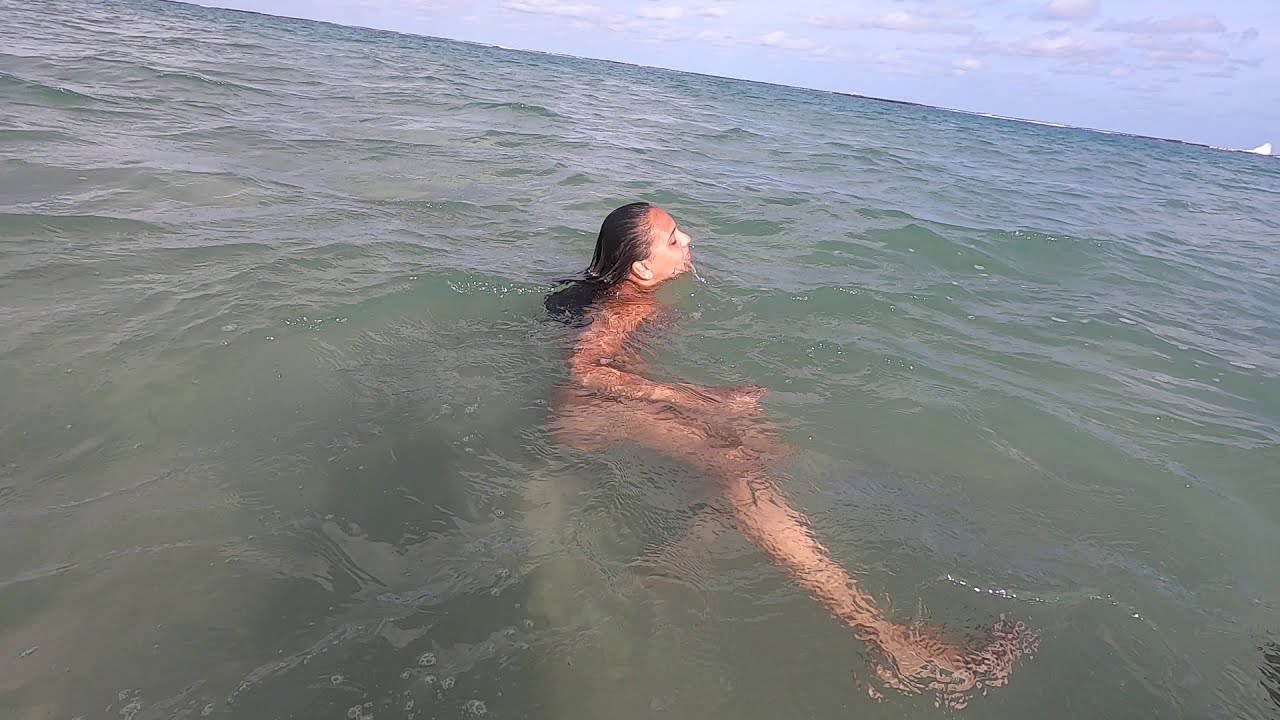In this highly detailed and vivid landscape photograph, a woman is seen swimming in the ocean, primarily submerged in the murky, greenish-brown water that transitions to a clearer blue as it nears the horizon. Her long, slicked-back brown hair trails into the water, and only her head and parts of her arm and leg break the surface. She appears to be treading water or floating calmly, with her eyes closed. The sky above is mostly blue with a few scattered clouds. In the distance, towards the top right of the image, a small white object can be discerned, possibly a sailboat or a building on a distant shore. The sandy bottom is faintly visible through the somewhat opaque water, suggesting she is in relatively shallow waters. Her skin tone appears olive, hinting that she could be Latina, Middle Eastern, or a tanned Caucasian. The overall scene captures a serene moment of solitude and relaxation in a vast body of ocean water, likely near a beach.